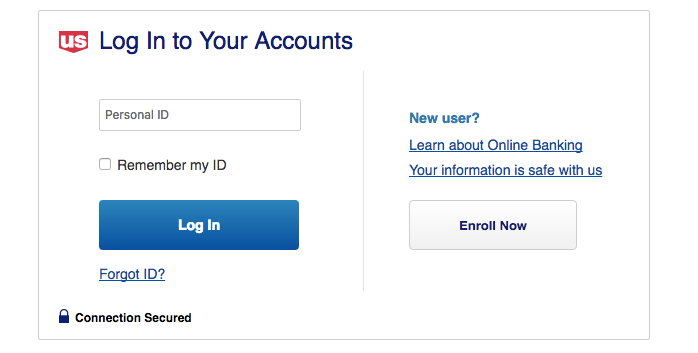In this image, we see a user interface for a login page encased in a gray-outlined rectangle. Located in the upper left corner is a logo featuring the letters "US" in bold white block text, surrounded by red. To the right of this logo, a statement in bold black print reads, "Log in to your accounts."

Below this statement is an open text box labeled "Personal ID." Adjacent to it, on the right, is a small square checkbox with the option to "Remember my ID." Beneath these fields is a blue action button labeled "Log in."

Further down, there is a blue hyperlink reading "Forgot ID?" with a question mark. In the lower left corner of the image, an icon of a lock is displayed alongside the text "Connection secured."

On the right side of the image, blue text introduces the section with "New user?" followed by the underlined prompt "Learn about online banking." It is accompanied by an assurance that "Your information is safe with us." Directly below these statements is a white action button that reads "Enroll now."